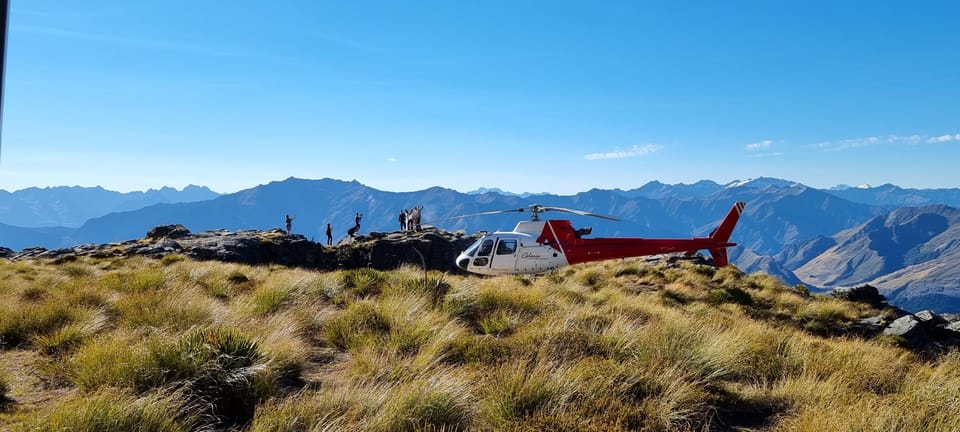The photograph captures a striking scene of a red and white helicopter, either landing or preparing for takeoff, positioned on a grassy mountaintop under a bright cyan blue sky with wispy clouds. The helicopter, with its stationary propellers, is primarily white at the nose and red at the midsection and tail. Surrounding the helicopter is a mix of light green and brown grass, illuminated by the sun, which creates a spectrum of yellow and green tones across the pasture.

In the foreground, a rocky cliff edge borders the grassy area, where a group of seven individuals is gathered. Three figures are prominently highlighted: one person standing away from the group with outstretched arms, another sitting centrally and gazing at the expansive blue-gray mountain range ahead, and a third individual standing nearby, also looking towards the mountains. The remaining members of the group are bunched together, similarly extending their arms, perhaps indicating some involvement in a coordinated effort. The thick foliage near the left side of the image complements the thinner vegetation closer to the helicopter, adding depth to the scenic landscape.